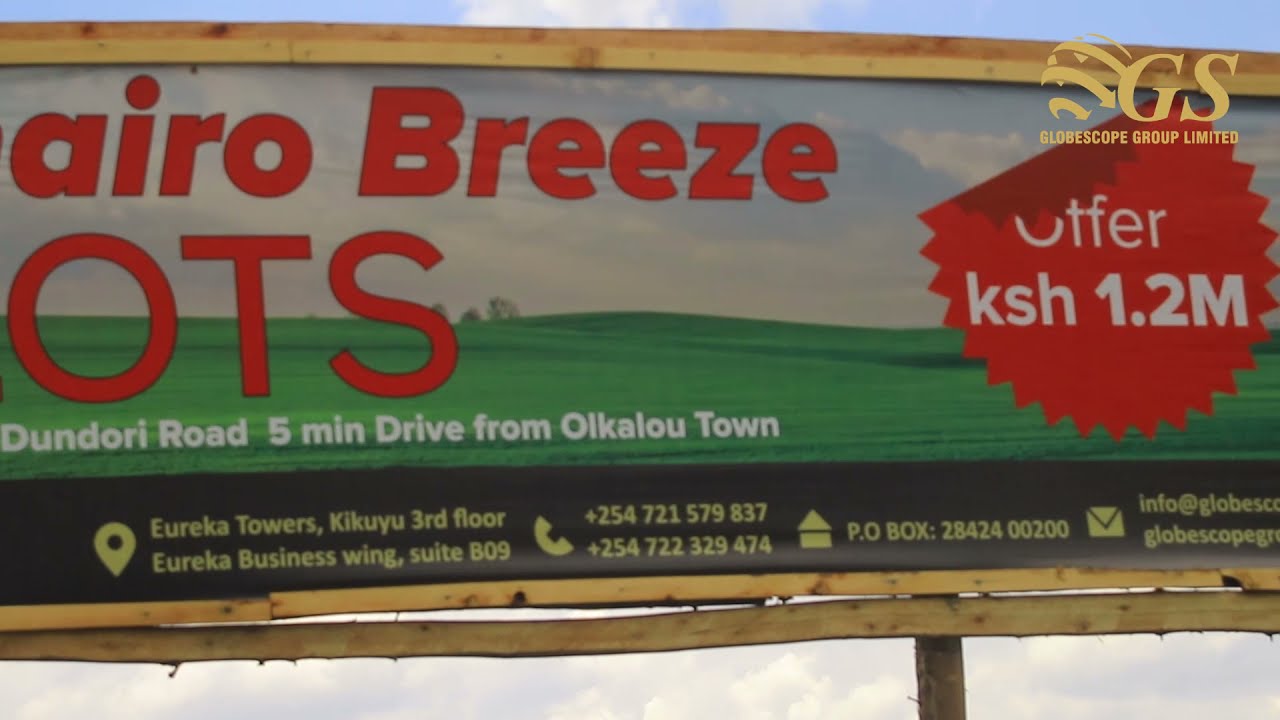The image features an outdoor billboard supported by a rugged wooden frame and a visible wooden post at the bottom right. In the top right corner of the billboard, there's a logo for Globe Scope Group Limited, consisting of a globe encircled by yellow arrows and the bold, golden letters 'G' and 'S'. The billboard itself showcases a lush, green landscape under a clear blue sky. The main text in red says "Cairo Breeze OTS" (the "C" is partially cut off). Beneath this, in white text, it reads "Dundori Road, 5-minute drive from Olkalao Town." A red sunburst-shaped sticker on the right side advertises, "Offer KSH 1.2 M." Lower on the billboard, details are provided in black text: "Eureka Towers, Kikuyu, 3rd Floor, Eureka Business Wing, Suite B09," followed by two phone numbers: "+254 721 579837" and "+254 722 329 44474," a P.O. box number "2842400200," and partially visible email addresses starting with "info@globe" and "globescopegr."